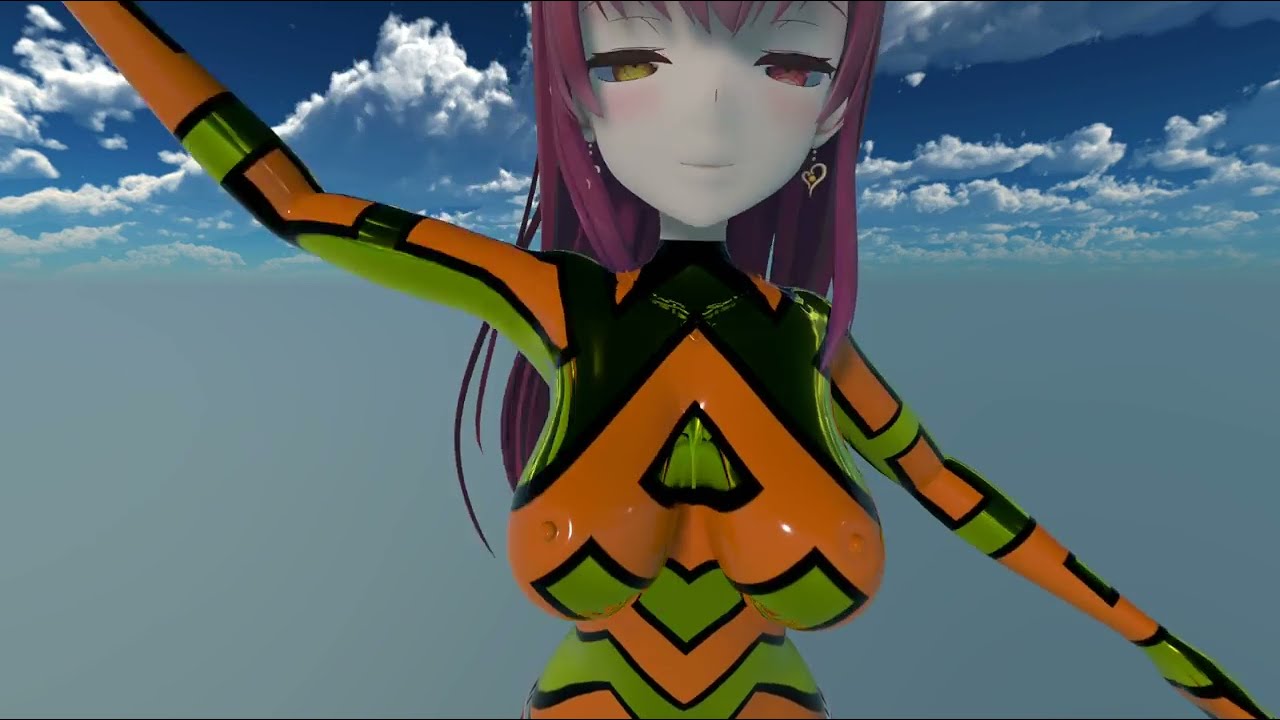This horizontal rectangular image depicts an anime-style doll held up against a backdrop of blue sky and dark clouds. The doll has a distinctly unrealistic, almost ceramic appearance, with an outfit in vibrant orange and green hues. Added details include black stripes and possibly orange earrings shaped like hearts, which complement her exaggerated, stylized features. Her prominent breasts and narrow waist are accentuated by the tight-fitting outfit. She has an unmistakable white face with large, elaborate eyes—one green and one pink—and her hair cascades down in a reddish-brown hue past her chest. Despite her very thin arms being visible, her hands are not, as they extend in opposite directions. The overall scene conveys a surreal, painted quality, juxtaposed with the doll's starkly realistic details against the backdrop of the open sky.